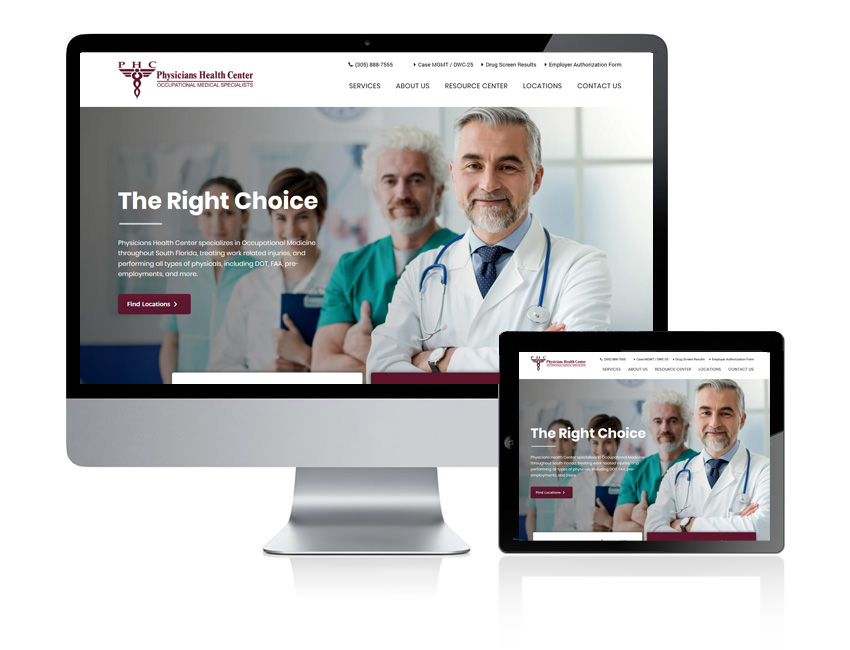The advertisement for the Physician's Health Center depicts a modern approach to healthcare services. Set against a pristine white background, the focal point is an unusual computer monitor with a wide horizontal screen that is notably short in height. Below this monitor, the same screen image is replicated on a horizontally positioned black smartphone, demonstrating the center's digital accessibility.

At the top, the logo of the Physician's Health Center is prominently displayed in red, accompanied by the center's phone number in gray. Above the images, the website's navigation headers include "About Us," "Resource Center," "Locations," "Contact Us," and other small-print links, one of which seems to be "Employer Authorization Form."

The core message of the ad, "The Right Choice," is highlighted along with a call-to-action in a red box stating "Find Locations." Although difficult to read due to small font size, the advertisement includes additional text that elaborates on the center's offerings.

On the screens, viewers can see an image of four diverse medical professionals, featuring:
1. A gentleman in a white lab coat with a stethoscope, wearing a shirt and tie, positioned at the forefront with his hands folded.
2. A male doctor in green scrubs.
3. A female doctor in a white coat holding a medical chart.
4. Another individual in green scrubs, standing furthest back on the left.

Together, these elements emphasize the center's comprehensive and professional healthcare services, making "Physician's Health Center: The Right Choice" their clear, confident message.